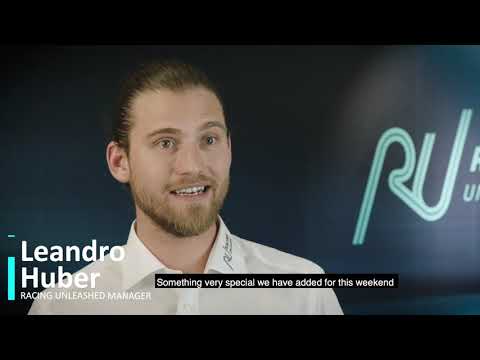The image is a detailed still from an interview featured in what appears to be a YouTube video. The subject is a young white man named Leandro Huber, as indicated by the on-screen text overlay identifying him as the "Racing Unleashed Manager". He is in mid-sentence, with his mouth open, revealing his teeth. Leandro has a reddish-brown beard and matching slicked-back hair that appears to be pulled into a bun. His attire consists of a white button-down shirt, which displays black writing on the collar. 

Leandro's facial expression is animated, with wide eyes that give him a joyous, engaged demeanor. The background behind him is a gradient of dark grayish-blue on the right, with parts of a stylized logo visible, including the letters "R" and "U" in teal. The top and bottom of the image are partially blocked by black rectangles. The bottom rectangle houses closed captioning text that reads, "something very special we have added for this weekend," indicating the context of his speech.